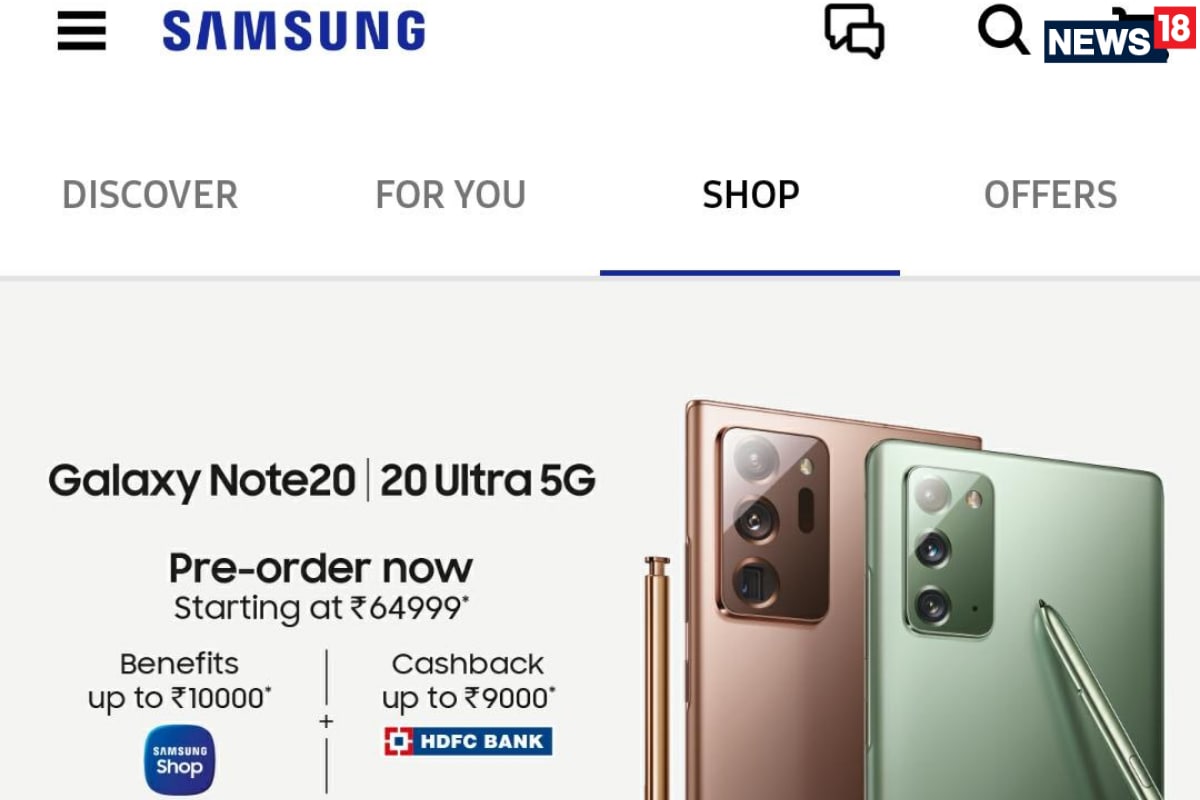This image captures the Samsung Store webpage. At the top left, there is a menu button represented by three black lines. Adjacent to this on the right is the Samsung logo in a deep navy blue color. On the far right, there is a chat icon with two chat bubbles, followed by a search icon, and then the text 'News 18'. 

Beneath this header section, there are four tabs labeled: Discover, For You, Shop, and Offers. Below these tabs, there is a prominent advertisement for the Samsung Galaxy Note 20 and Note 20 Ultra 5G, which invites viewers to pre-order now starting at ₹64,999, accompanied by an asterisk.

At the bottom left corner of the advertisement, it mentions benefits up to ₹10,000, while on the bottom right, it highlights a cashback offer up to ₹9,000 from HDFC Bank. The text 'Samsung Shop' appears on the left side.